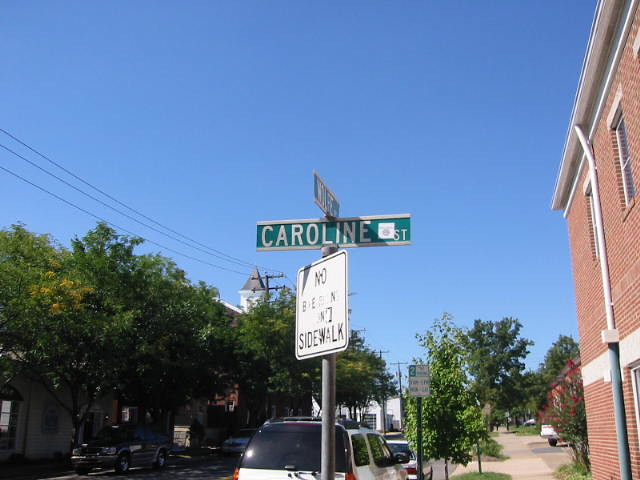This photograph captures a detailed scene at the intersection of Caroline Street and an unidentified cross street, whose name is not readable from the angle of the shot. Centered prominently is a green street sign with white text for Caroline Street. Below it, a white sign with partially legible text reads "No something something sidewalk." Further down the street, a two-hour parking sign is visible. The street is flanked by cars parked on either side and lined with numerous trees, particularly on the left side. To the right of the image, there's a brick building with a visible drain spout running along its side. In the distant background, a structure resembling a clock tower or church steeple rises against a clear blue sky, which is unmarred by clouds. Utility lines stretch along the left side of the image, adding to the suburban atmosphere. The main focus is on the street sign, highlighting the intersection of Caroline Street in this quiet, sunny neighborhood.